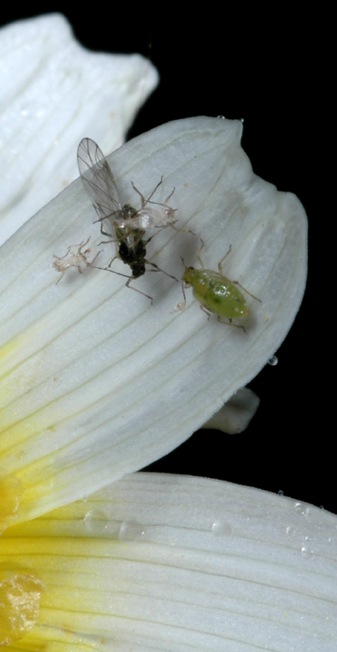This detailed photograph captures a realistic scene of several insects on a delicate white and yellow flower. The image, vertically oriented at about two and a half to three times as tall as it is wide, prominently features a large petal angling upward and to the right, with thin gray seams running horizontally along its surface. This particular petal is the focus, hosting several insects. 

On the petal, there's a notable light green bug, oval-shaped with a shell-like body adorned with darker green spots. This bug has six legs. Above it hovers a black-headed mosquito-like insect with transparent wings, distinct with visible veins and also possessing six legs. Additionally, the image reveals one or two very tiny, almost translucent insects on the same petal.

The backdrop of the flower includes three prominent white petals, especially visible on the left-hand side, with hints of yellow from the flower’s center in the bottom left corner of the image. Small droplets of moisture add a touch of realism, glistening on the surfaces of the petals. The background of the photograph transitions into a stark black on the upper right and right side, emphasizing the intricate details of the flower and the bugs against the dark contrast.